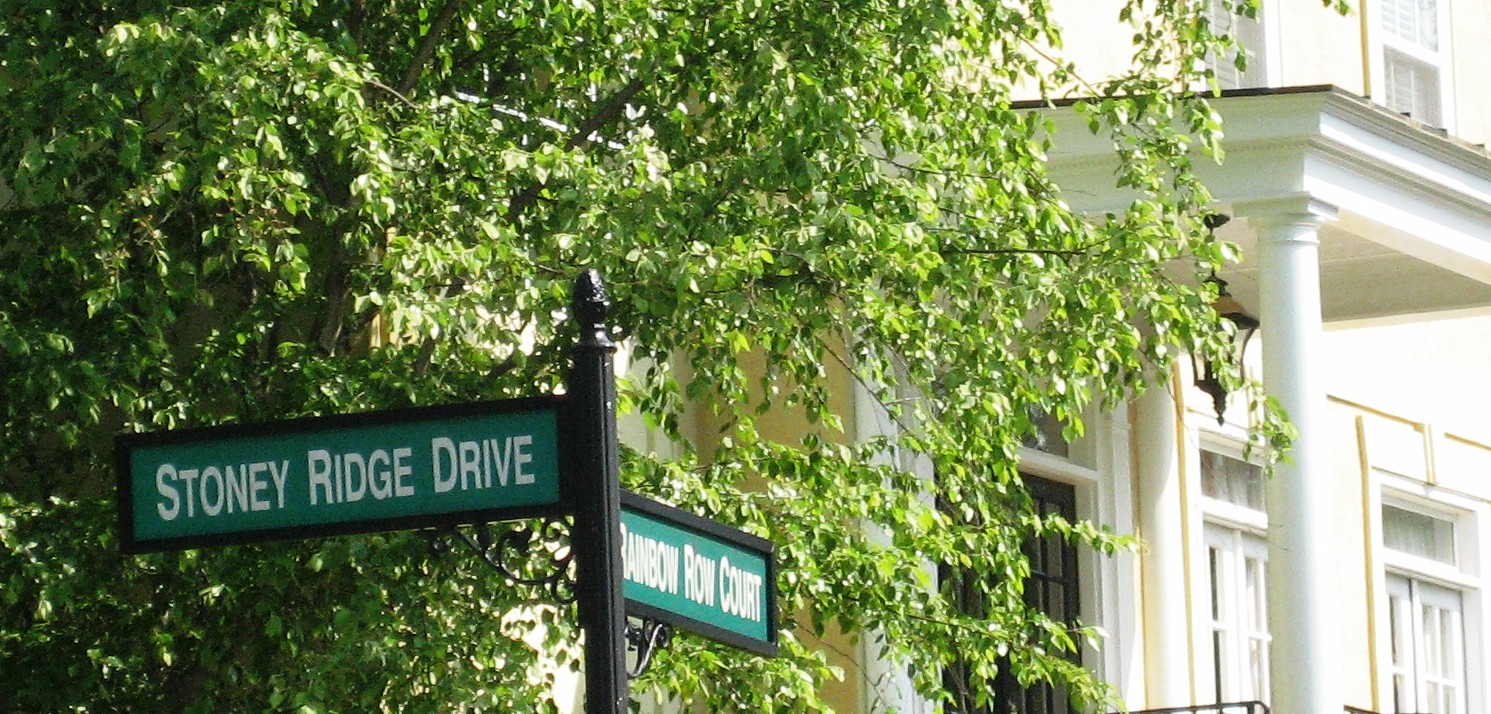In this image, we are presented with a close-up view of a black, metallic street sign situated in front of a multi-level house. The street sign features two green plaques with white lettering, each pointing in different directions, indicating "Stony Ridge Drive" and "Rainbow Row Court." The sign stands before a charming yellow-painted house, most of which is obscured by a large, verdant tree with small, vibrant green leaves. Though the lush foliage partially conceals the residence and even slightly obscures the sign, we can still discern some architectural features: the house boasts an inviting porch supported by white pillars and is adorned with several windows—three on the main floor and two on the floor above. The focal point of the photograph is clearly the street sign, with its stark black and green contrasting against the leafy backdrop, offering an intriguing glimpse into this picturesque neighborhood scene.